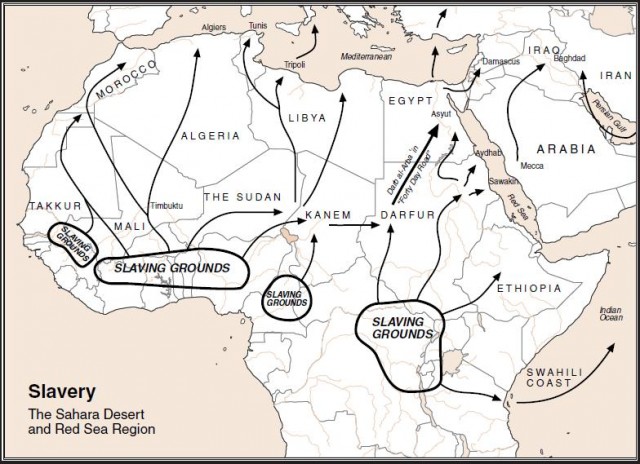This image is a detailed, two-toned map of Africa and the surrounding regions, with a light pinkish background for the seas and a white background for the landmasses. The map is titled "Slavery, The Sahara Desert, and Red Sea Region" at the bottom left in dark blue letters. It outlines and labels countries with sparse lines in dark blue. The prominent feature of this map is the numerous black arrows originating from circled areas labeled repeatedly as "slaving grounds." These arrows point towards various destinations across the map.

Countries and regions identified as slaving grounds include Morocco, Algeria, Libya, Egypt, Ethiopia, Darfur, Sudan, Mali, and the Swahili Coast. Arrows extend to farther regions in the Middle East, including Iraq, Iran, Tripoli, and Damascus. The map emphasizes the historical trade routes of slavery with extensive arrow paths leading from these slaving grounds to different points both within Africa and extending into the Arabic Peninsula and beyond.